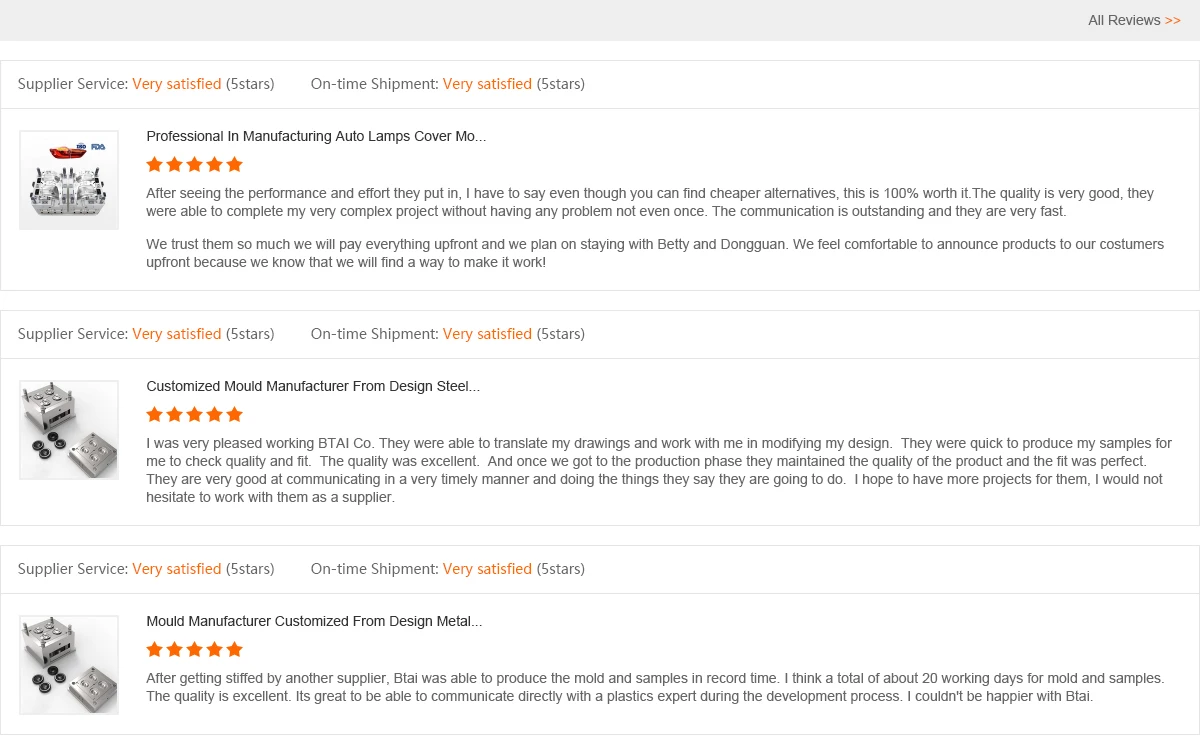This screenshot showcases a white page with a light gray bar at the top. Positioned all the way to the right, the text "All Reviews" suggests it's a review section for a specific service. The reviews have been filtered by two categories: "Supplier Service" and "On-Time Shipment," both marked as "Very Satisfied" with a five-star rating. 

There are three reviews visible, each sharing commonalities and a perfect five-star satisfaction rating for both shipment and supplier service. 

1. The first review focuses on "Professional and Manufacturing Auto Lamps Cover" and includes a unique picture, indicating the purchase of a distinct item from other reviews.
2. The second review describes "Customized Mold Manufacturer from Design Steel."
3. The third review also addresses a "Mold Manufacturer" but specifies the material as "Design Metal."

Interestingly, the second and third reviews appear nearly identical in content and imagery, differing only in the order of their names.

All reviewers express high levels of satisfaction with products from the supplier, BTAI Company. The individual experiences and visual elements suggest positive feedback for both the distinct and similar items offered by the supplier.